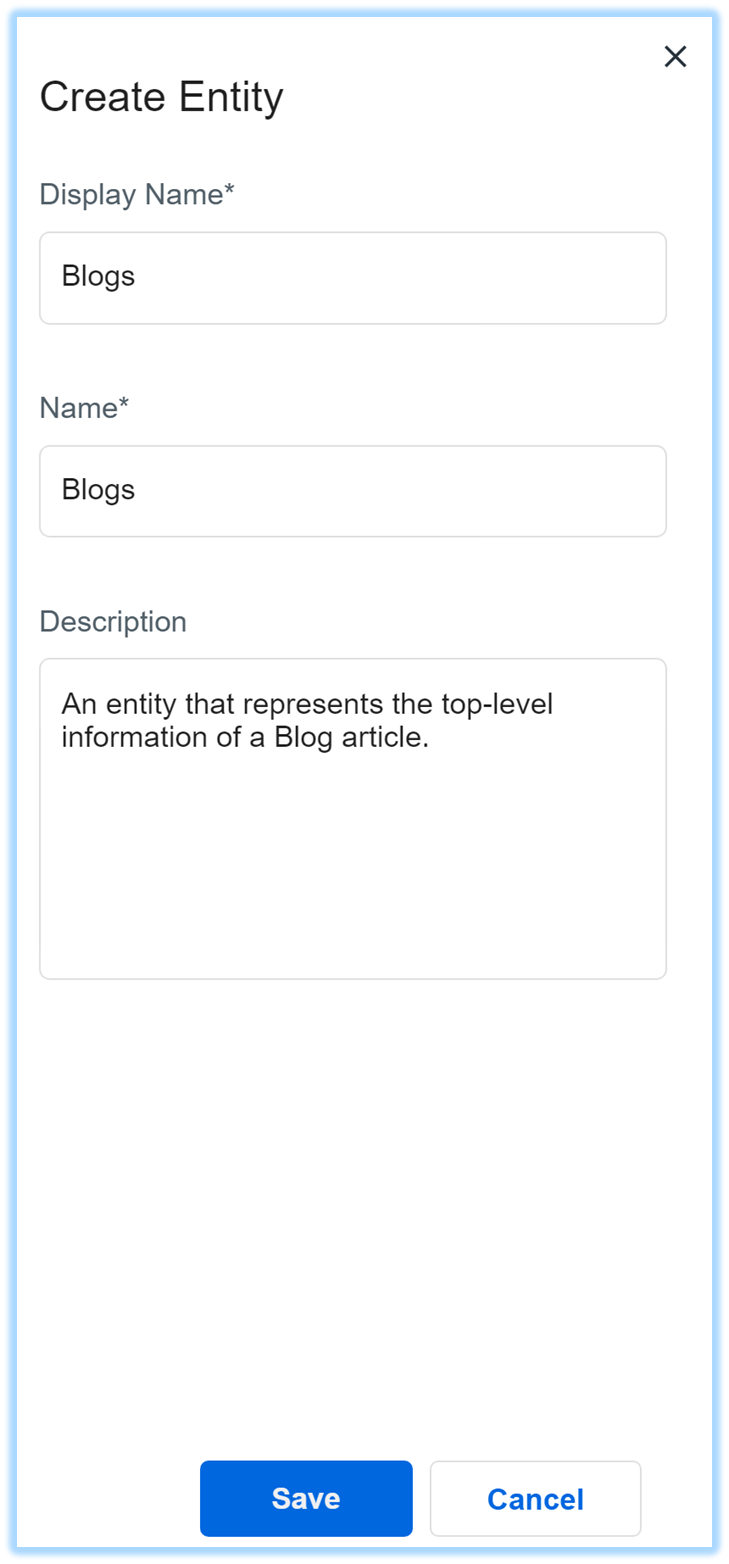A screenshot displays a pop-up window from an application or website, outlined in light blue. The background of the pop-up is white, with dark gray text for labels and fields. In the top right corner, there's an "X" button to close the pop-up. The pop-up is titled "Create Entity."

Below the title, the label "Display Name" appears, marked with an asterisk to indicate it's a mandatory field. The field is filled with the word "Blogs." The next label, "Name," also mandatory and marked with an asterisk, is similarly filled with the word "Blogs."

Further down, there is a textbox under the label "Description." Within this field, the following text is entered: "An entity that represents the top-level information of a blog article."

At the bottom of the pop-up, there are two buttons. The left button is blue and labeled "Save," while the right button is white with blue text that reads "Cancel."